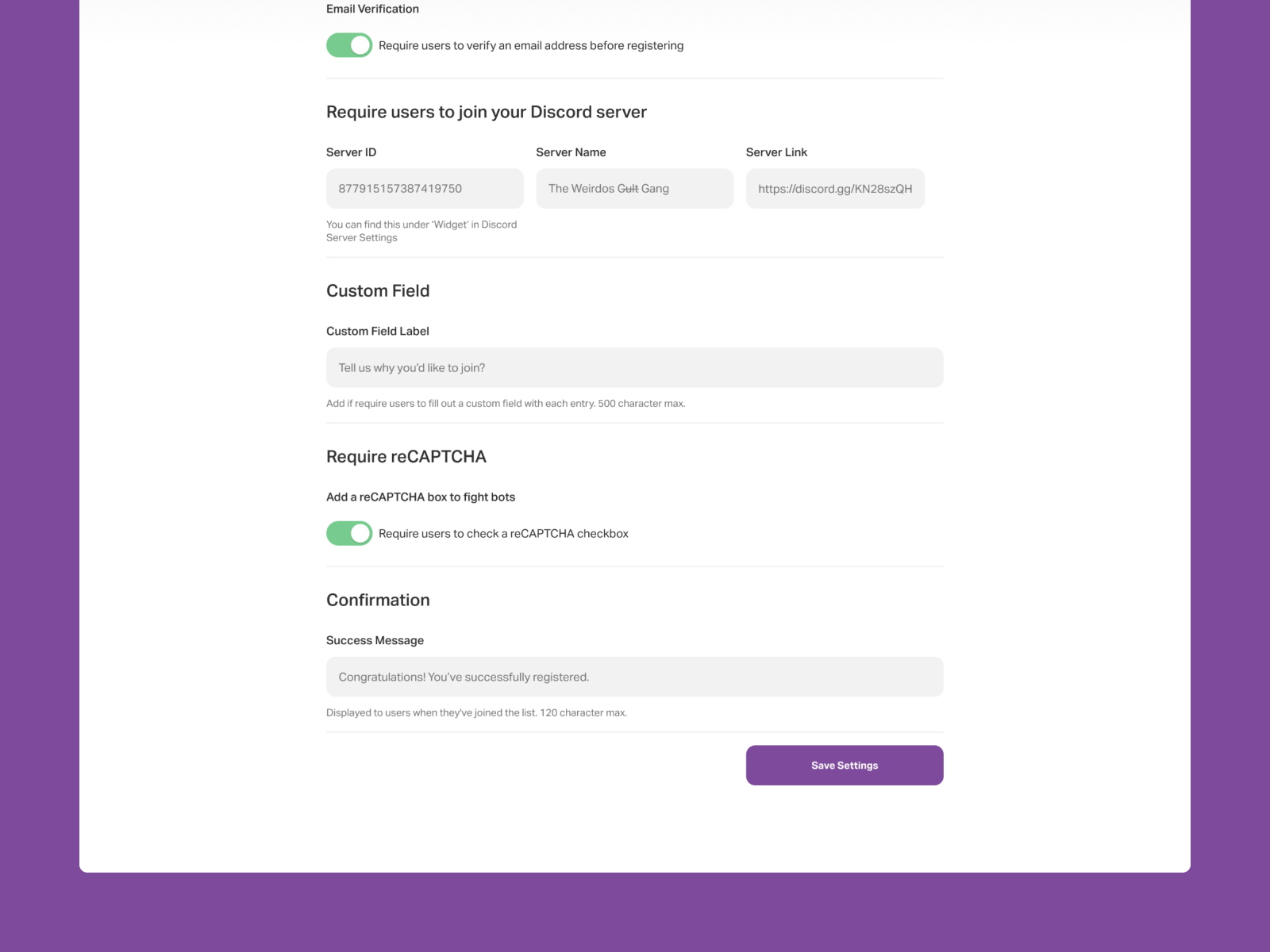**Settings Page Overview:**

1. **Email Verification**
   - **Status:** Enabled
   - **Description:** Requires users to verify their email address before registering.

2. **Discord Server Requirement**
   - **Option:** Require users to join your Discord server
   - **Server ID:** 877-915-1578 or 738-74-19750
   - **Server Name:** TheWeirdosCultGang
   - **Server Link:** [https://discord.gg/KN28szQH](https://discord.gg/KN28szQH)
   - **Description:** You can find this under the widget in the Discord server settings.

3. **Custom Field**
   - **Label:** Tell us why you'd like to join
   - **Description:** Requires users to fill out this custom field with each entry (500 character max).

4. **reCAPTCHA**
   - **Status:** Enabled
   - **Description:** Adds a reCAPTCHA checkbox to fight bots, requiring users to check it.

5. **Confirmation**
   - **Success Message:** Congratulations. You've successfully registered.
   - **Description:** This message is displayed to users when they successfully join the server.

6. **Save Settings**
   - Allows users to save any changes made on the settings page.

Overall, the settings page ensures security through email verification and reCAPTCHA, while fostering community engagement by requiring users to join a specified Discord server. The inclusion of a custom field allows for personalized user input.